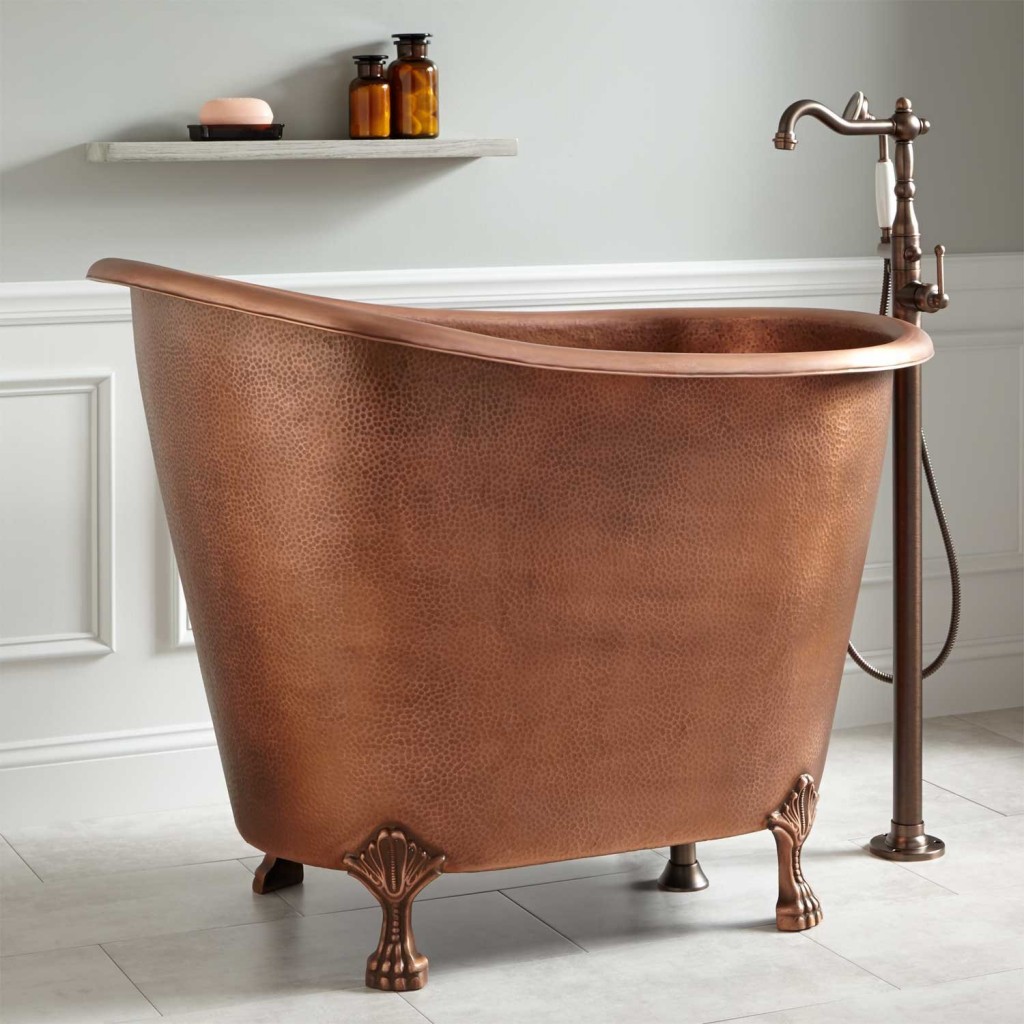The image depicts a freestanding deep bronze bathtub, sitting on copper feet, positioned against a backdrop of long rectangular white tiles. A tall brass spout, extending from the floor to over the tub, provides a striking focal point. The wall above the white tile border features a light gray finish, accented by an oversized white trim. A floating white shelf is mounted on the back wall, holding brown bottles with cotton balls inside and a pink bar of soap on a bronze glass soap tray. The lighting in the room comes from the right, casting a soft glow over the bathtub and its surroundings.